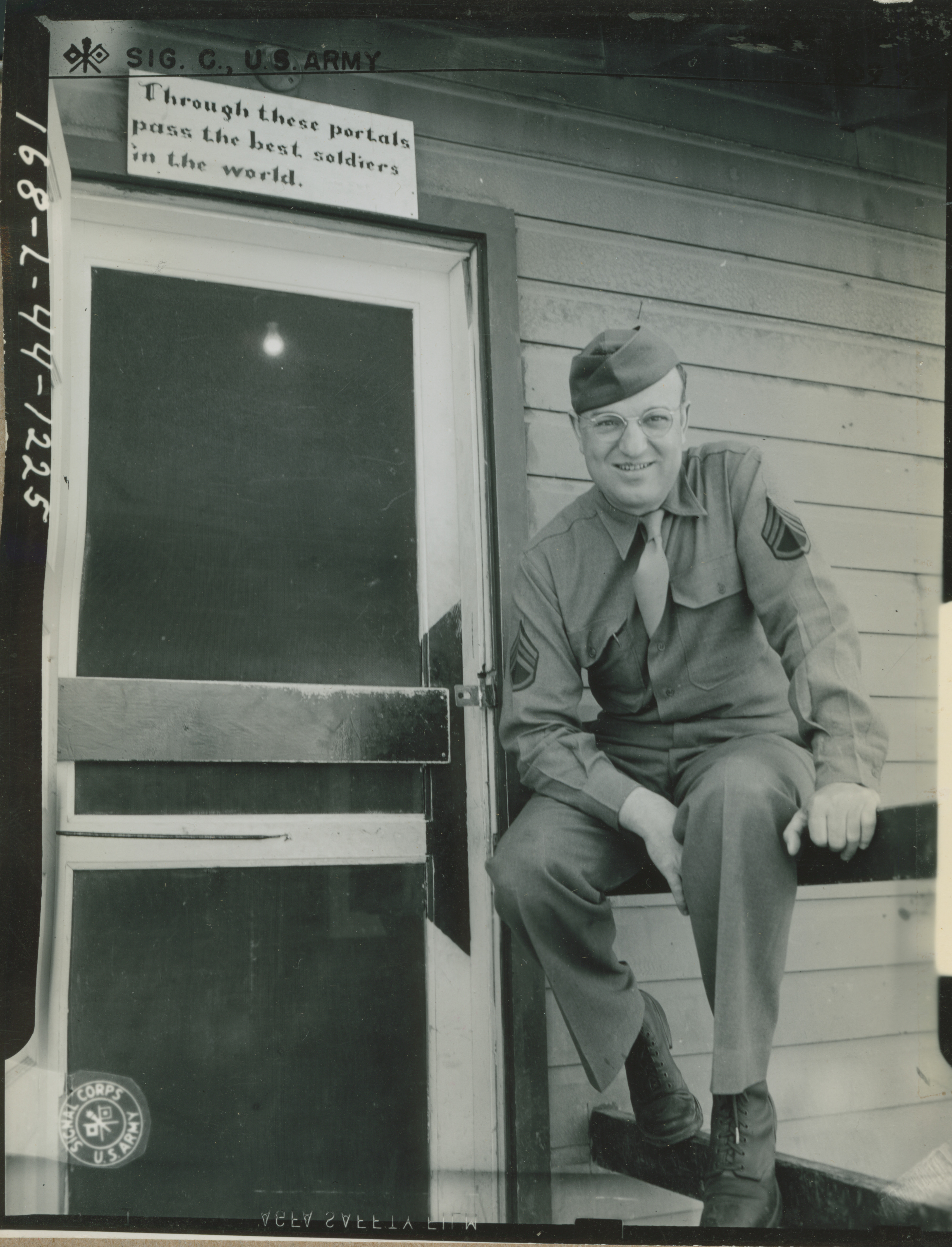This black-and-white photograph likely dates back to the Second World War and features a soldier in his late 20s, dressed in full military uniform. The man, presumably a sergeant given the insignias on his shoulders, sits on a fence outside a barracks or mess hall on a military base. His uniform includes a long-sleeved shirt, a tie, standard GI boots, and a cap, complemented by his glasses. He sports a subtle, half-smile. Beside him, a screen door and a prominent sign reading, "Through these portals pass the best soldiers in the world," are visible. Additional details include a unique white door with the number "NA 1687441225" and a small logo. The building's wooden structure adds to the historical ambiance of the image.